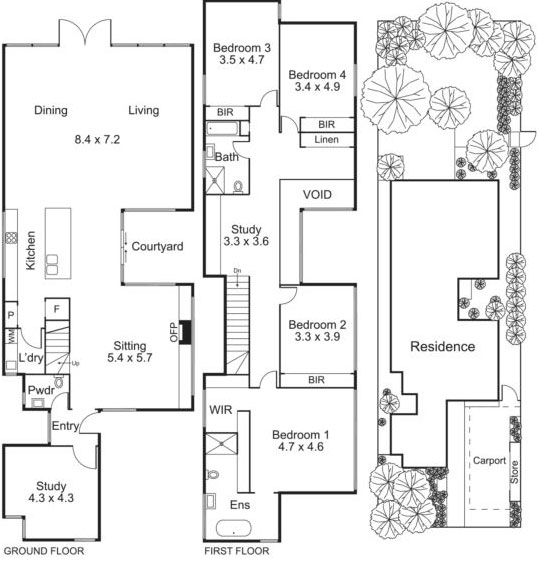A detailed bird's-eye view blueprint of a house rendered in black and white. The blueprint meticulously outlines the exterior walls, individual rooms, and all major furniture placements. The black lines sharply contrast against the white background, creating a clear visual separation. Each room is labeled with its function in black text, including the dining and living room (8.4 x 7.2 meters), Bedroom 1 (4.7 x 4.6 meters), Bedroom 2 (3.3 x 3.9 meters), Bedroom 3 (3.4 x 4.9 meters), and Bedroom 4 (3.5 x 4.7 meters). Additional spaces such as the sitting area, study, residence, carport, and store are also distinctly marked. The blueprint includes structural elements spanning the first and ground floors, with designated entry points. Outside, the aerial view captures outdoor elements like umbrellas and vegetation, possibly bushes or trees, illustrated in black and white with flower-shaped patterns. Every detail is meticulously outlined in black and white, giving a comprehensive overview of the house layout and its surroundings.